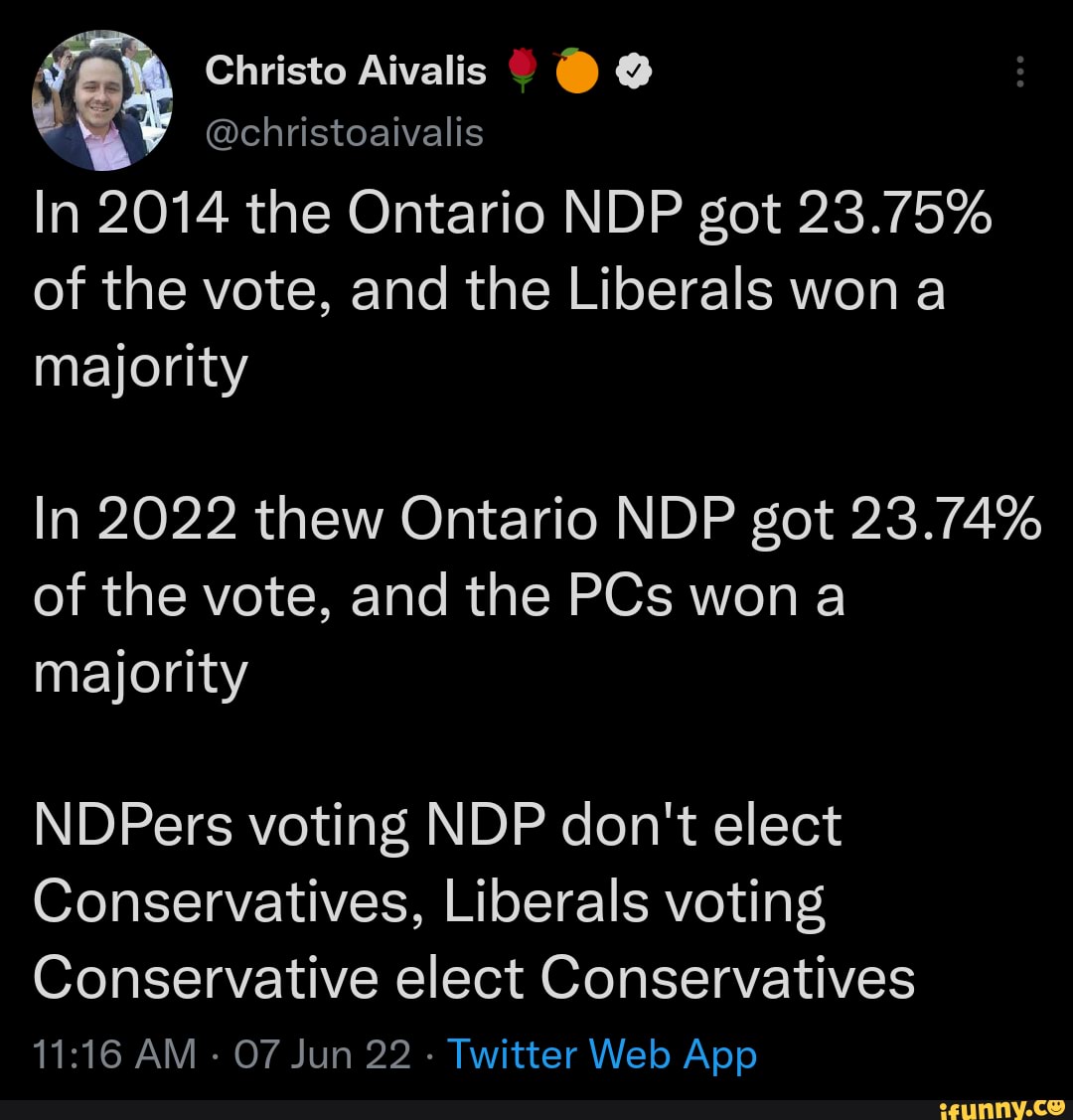This detailed screenshot captures a Twitter post viewed through the Twitter web app interface, distinguished by its dark mode setting, with a black background. The tweet is authored by Cristo Avalis, whose profile name is accompanied by a series of unique icons—a rose, an orange, and a checkmark with a cloud. The tweet's content is presented in a larger font and reads as follows:

"In 2014, the Ontario NDP got 23.75% of the vote and the Liberals won a majority. In 2022, the Ontario NDP got 23.74% of the vote and the PCs won a majority. NDPers voting NDP don't elect conservatives; liberals voting conservative elect conservatives."

The timestamp below the tweet indicates it was posted at 11:16 AM on June 7, 2022. The phrase "Twitter web app" at the bottom signifies the platform used to publish the tweet, displayed prominently in blue text.